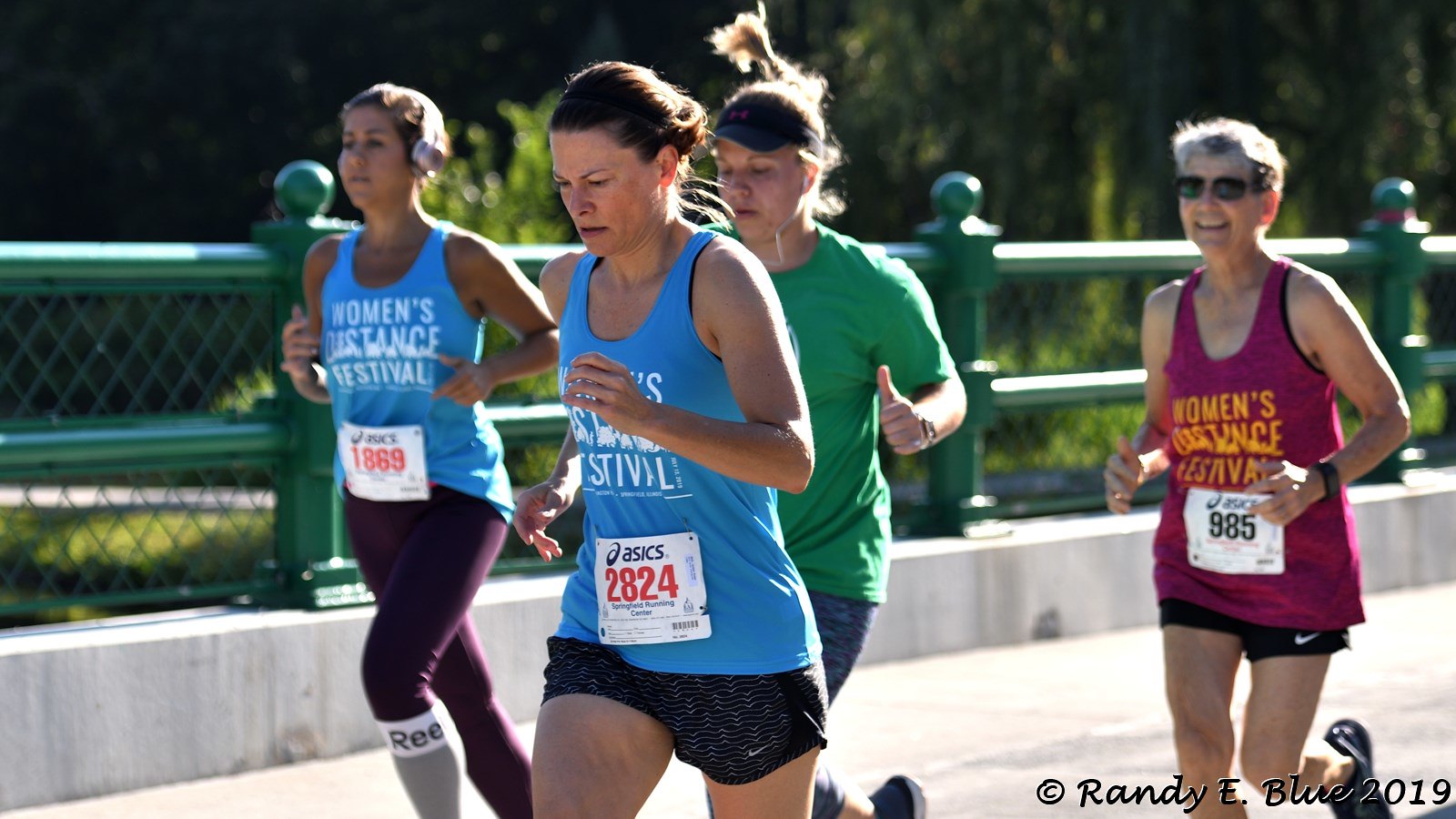The image captures an ongoing long-distance foot race, comprising exclusively of women participants, judging by the relaxed expressions indicative of an endurance event. They're running on a bridge, evidenced by the green railing and concrete structure, set against a backdrop of trees. 

Leading the pack are two women in identical blue tank tops. The woman in the center dons black shorts and bears the number 2824 while to her left is another young woman, wearing blue sleeveless shirt and headphones, numbered 1869. Accompanying them is a participant in a green T-shirt with blue tights, distinguished by her hat, running slightly behind. Further back, an older lady, likely a senior citizen, is notable with her glasses and burgundy T-shirt, numbered 985, paired with black shorts and smiling as she runs. Each shirt bears the inscription "Women's Distance Festival" indicating the event's theme. 

In the background, a green barrier fence can be seen, reinforcing the race setting. At the bottom right of the image, a watermark reads "© Randy E. Blue, 2019," marking the photo's credit.